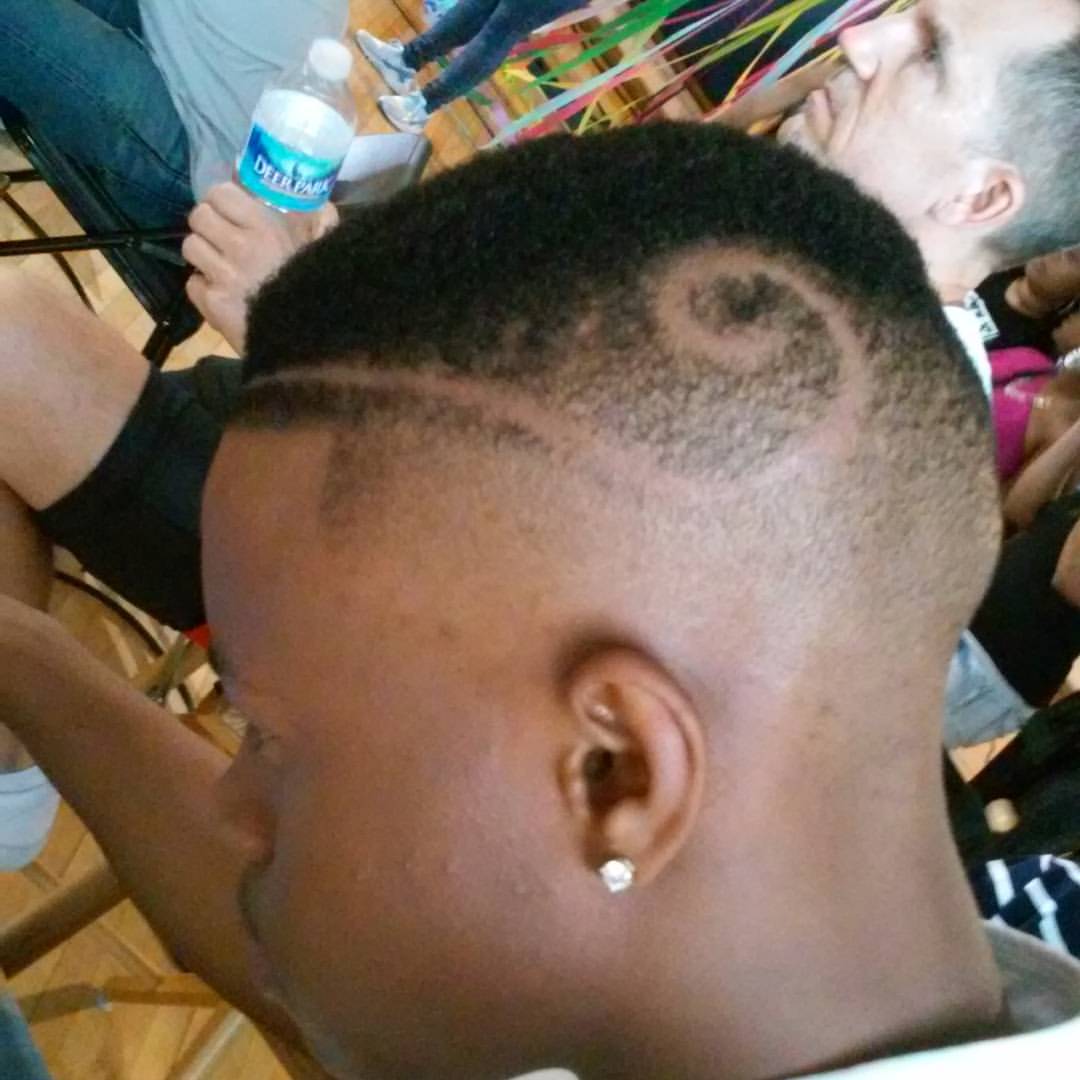The image is a close-up photograph of the back of a man's head. The man, likely African-American, has short, curly black hair with a swirl pattern cut into the side. He is wearing diamond-studded earrings. The man is looking down at the ground, which is covered in white and tan-colored tiles. Next to him, another person, who appears to be older with short gray hair, is sitting. This person is wearing black shorts, white shoes, and a white polo shirt, and is holding a clear plastic bottle with a blue label that reads "Deer Park" and has a white cap. In the background, there are several people either sitting or standing, but they are mostly cut off at the edges of the photograph. The event seems to be taking place in a setting that might be a gymnasium, adorned with green, light blue, pink, and yellow streamers hanging above. The person with the black hair and brown skin is centered in the image, dominating the scene.